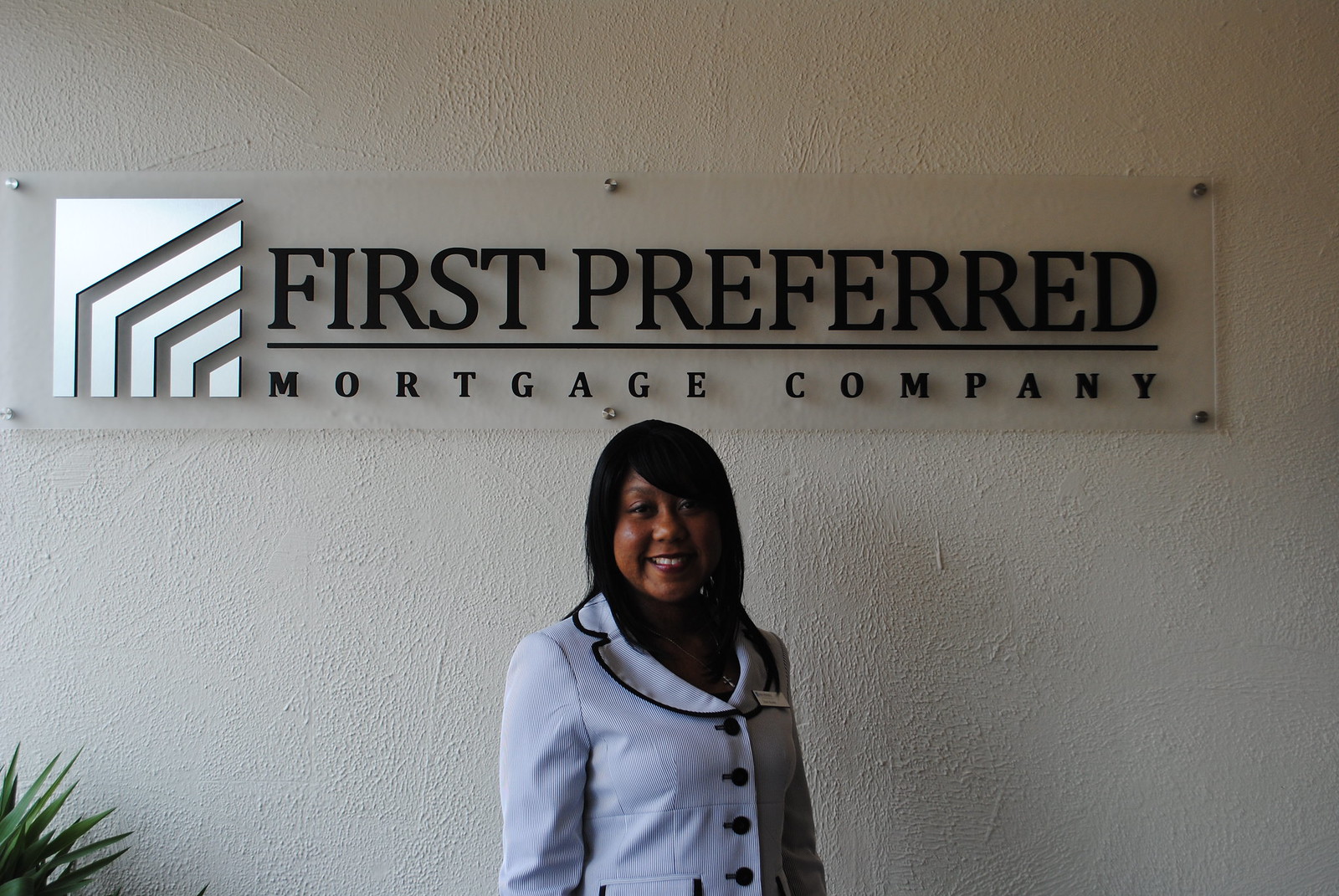A woman with black hair, who appears to be of African descent, is posing in front of a wall that features a sign. The sign prominently displays a silver logo on the left and the text "First Preferred Mortgage Company" on the right. The woman is standing directly beneath this sign, smiling warmly. She is wearing a white coat with black accents and a name tag, suggesting that she might be an employee of the company. The edges of a lush green plant are visible in the left-hand corner of the image, adding a touch of nature to the scene. The woman’s makeup is thoughtfully applied, complementing her professional appearance.